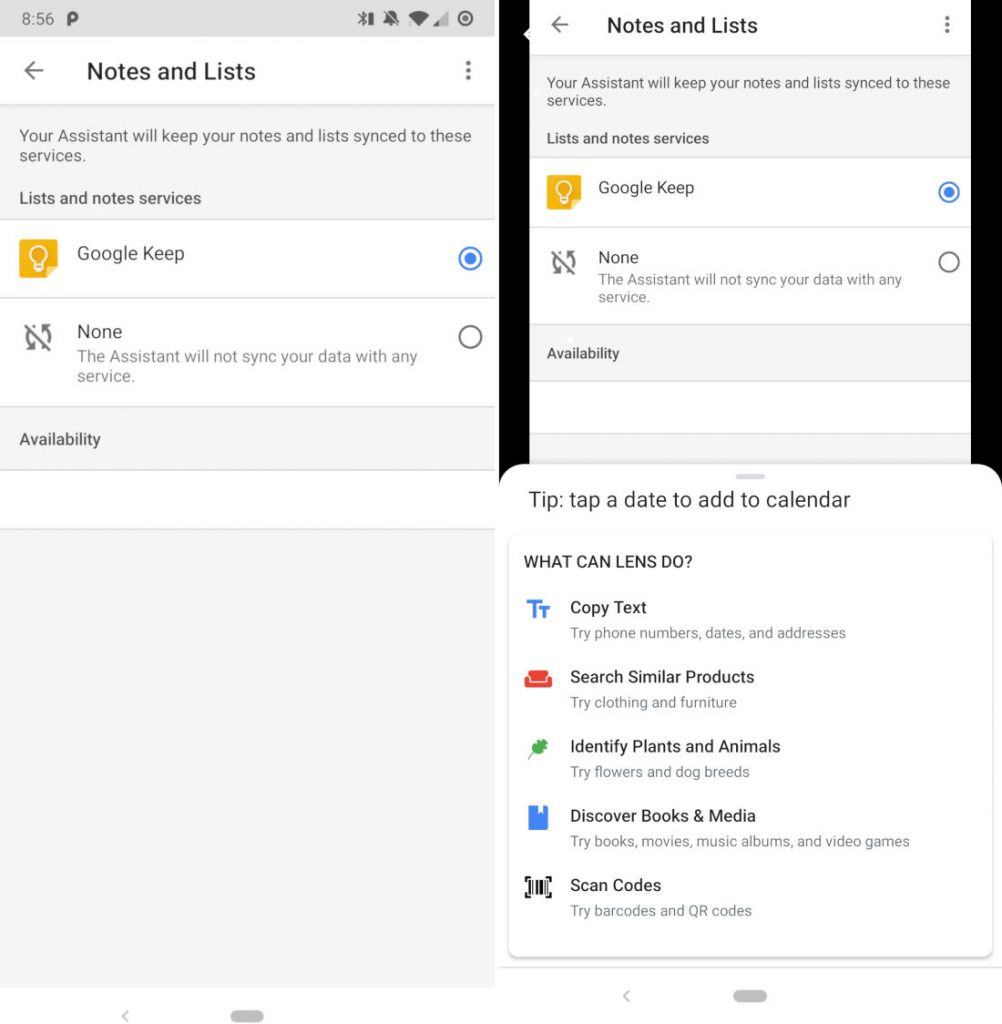Here is the cleaned-up and detailed caption for the image:

---

The image showcases multiple screenshots captured from a smartphone or tablet, displaying various interface elements and notifications. 

In the top left corner, the time is indicated as "0856" in military format, without specifying AM or PM. Adjacent to the time is a dark 'P' symbol. Following this is a series of icons: a Bluetooth symbol with a line through it, a bell icon that is dark black with a gray line through it, a fully black cell phone or Wi-Fi signal indicator, and a mixed black and gray cell phone signal icon located in the corner. Additionally, a black circle with a smaller medium dark gray circle inside it is visible.

Below these icons, the interface is divided into different sections. On the left-hand side, within a white rectangle, a dark gray arrow points left. Next to the arrow is bold black text that reads "Notes and List," followed by three ellipses on the right-hand side. 

Beneath this section is a medium gray rectangle containing black text that reads: "Your assistant will keep your notes and list synced to those services." Below this, in bold black text, it says "List and note services." An icon of an orange square with a white light bulb inside it represents Google Keep, accompanied by a blue circle. Below, there is a white rectangle with a dark gray refresh symbol with a line through it, labeled "None" in black. Underneath, in gray text, it states: "The assistant will not sync your data with any service," next to a white circle.

The left side features a dark gray bevel with black text that reads "Availability." Towards the center-right, another screenshot displays black bezels on both left and right sides. A dark gray arrow pointing left is at the center with text "Notes and List" in black. Dark gray ellipses follow on the right. The description about syncing notes and lists is repeated but within a dark gray rectangle, emphasizing "Your assistant will keep your notes and lists synced to those services" and "List and note services" in bold black text.

Within this section, similar interface elements are visible, including the Google Keep icon and another white rectangle with the refresh symbol labeled "None," repeated text, and availability options. 

On the left, a dark gray area with a small black bar beneath it appears. Adjacent to it on the right is a white rectangle containing the text: "Tip: Tap a date to add to calendar" in dark black. Below, a question in bold black asks, "What can Lens do?" followed by various options. Bold blue uppercase "TT" precedes "Copy text," with gray text advising to "Try phone numbers, dates, and addresses." A red couch icon next to bold black text "Search similar products” has gray text instructing to "Try clothing and furniture." 

Another section shows a green leaf icon next to bold black text "Identify plants and animals," and the gray suggestion to "Try flowers and dog breeds." There is a dark blue square with a portion cut out, labeled "Discover books and media" in dark black, and gray text: "Try books, movies, music albums, and video games." Lastly, a black QR code with corner pieces has bold text "Scan codes" with the gray suggestion: "Try barcodes and QR codes."